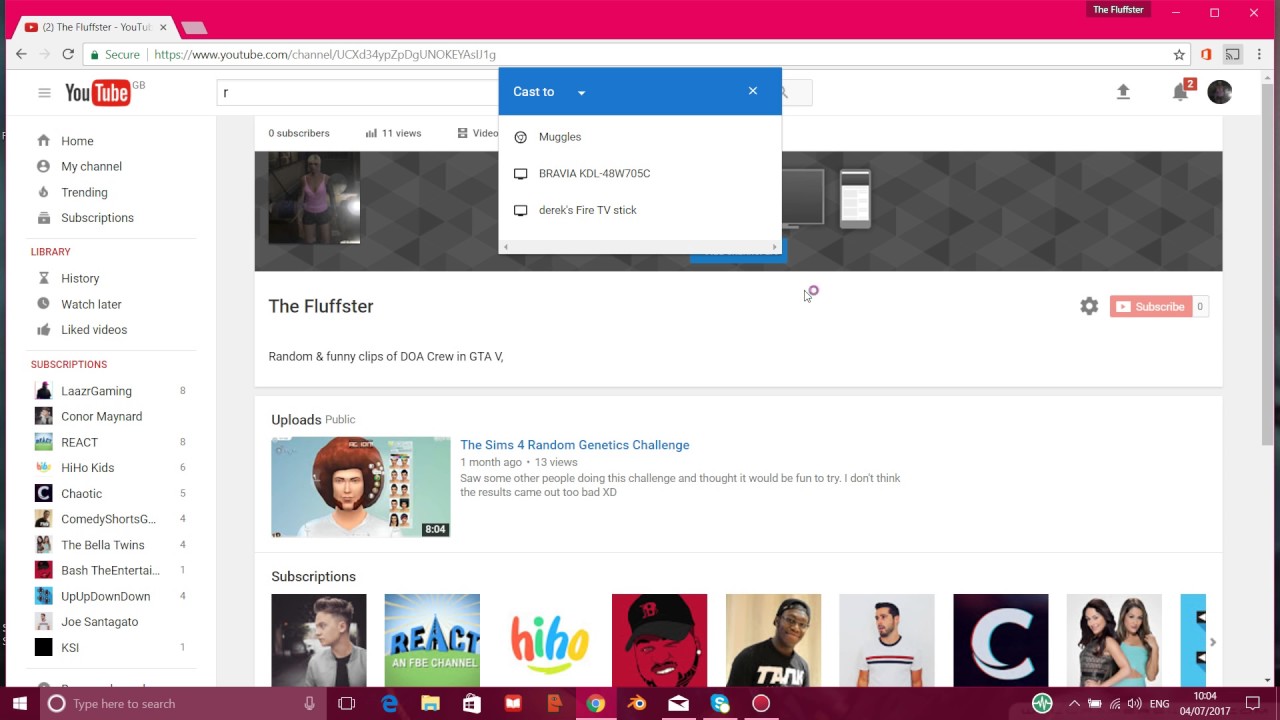The screenshot showcases a YouTube page open in a web browser on a Windows operating system. The browser window is defined by a rectangular layout. A reddish-pink bar stretches across the top of the window, containing a small clickable area with a brown background and white letters that read "the Fluffster." This element is situated to the left of the window control icons (minimize, maximize, and close).

The browser displays only one open tab labeled "the Fluffster on YouTube." A visible dropdown menu labeled "Cast To" offers two options for casting: "Muggles Bravia KDL-48W705C" and "Derek's Fire TV Stick," with no selection currently made. In the top right corner, there are two notification icons.

The main content showcases "the Fluffster" channel, described as featuring "random and funny clips of DOA crew in GTA V." Below this description, the channel has an upload titled "The Sims 4 Random Genetics Challenge - One Month Ago," which has garnered 13 views. The video thumbnail shows a person wearing some sort of helmet, and the video duration is 8 minutes and 4 seconds. The video's description mentions that the creator decided to try the challenge after seeing others do it and was pleased with the results.

On the left side of the page, a sidebar lists navigation options: Home, My Channel, Trending, Subscriptions, and under the Library section—History, Watch Later, and Liked Videos. Below these are subscriptions to various YouTube channels, which include Laser Gaming, Conor Maynard, React, HiHo Kids, Chaotic, Comedy Shorts, The Bella Twins, Bash, The Entertain, Something, UpUpDownDown, Joe Santagato, and KSI.

Under the video description, there is a section for subscriptions, displaying several channel icons. These include a man looking to the left, the "React" FBE channel, "HiHo," a man in a baseball cap, a person in a black t-shirt with "Tank" written on it, another individual in a white shirt with red and blue stripes and the letter "C," and two women.